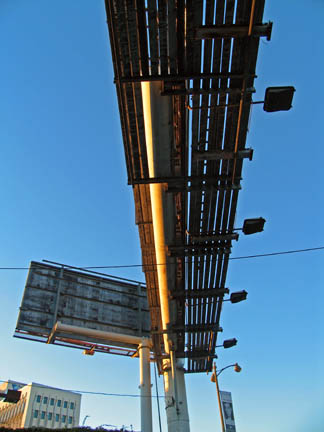The image captures a vertically-oriented, daytime scene viewed from the ground looking upwards beneath a billboard structure. The billboard, supported by a metal pole, is flanked by wooden scaffolding. Only the back side of the billboard is visible, with one vertical board and a horizontal board positioned further in the distance. Occupying the lower left corner of the frame is a beige and gold building with numerous windows, indicating at least three stories, although the bottom of the structure is not visible. A streetlight stands to the right of the billboard, contributing to the urban landscape captured in this photograph.